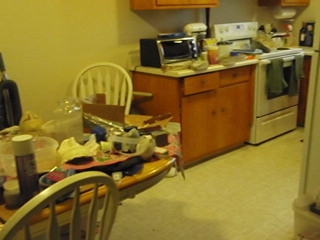A cluttered dining table takes up the foreground of this image, showcasing a farmhouse-style setup with a light wood-finished top and cream-colored sides, accompanied by two matching wooden chairs in cream. The table is strewn with various items, including a can of Aquanet hairspray, assorted dishes, bowls, and wrappers, creating a visibly chaotic scene. Beyond the table, the image transitions into a compact kitchen indicative of an apartment or small house, characterized by off-white linoleum floors and walls. The kitchen features medium-colored wooden cabinets, one of which supports a toaster oven surrounded by clutter. The white electric stove, visible in the background, has a couple of hand towels draped over its handle and is equally cluttered with miscellaneous items on and around it. In the bottom right corner of the image, the edge of what appears to be a refrigerator is partially visible, along with a glimpse of a square or rectangular-shaped container.